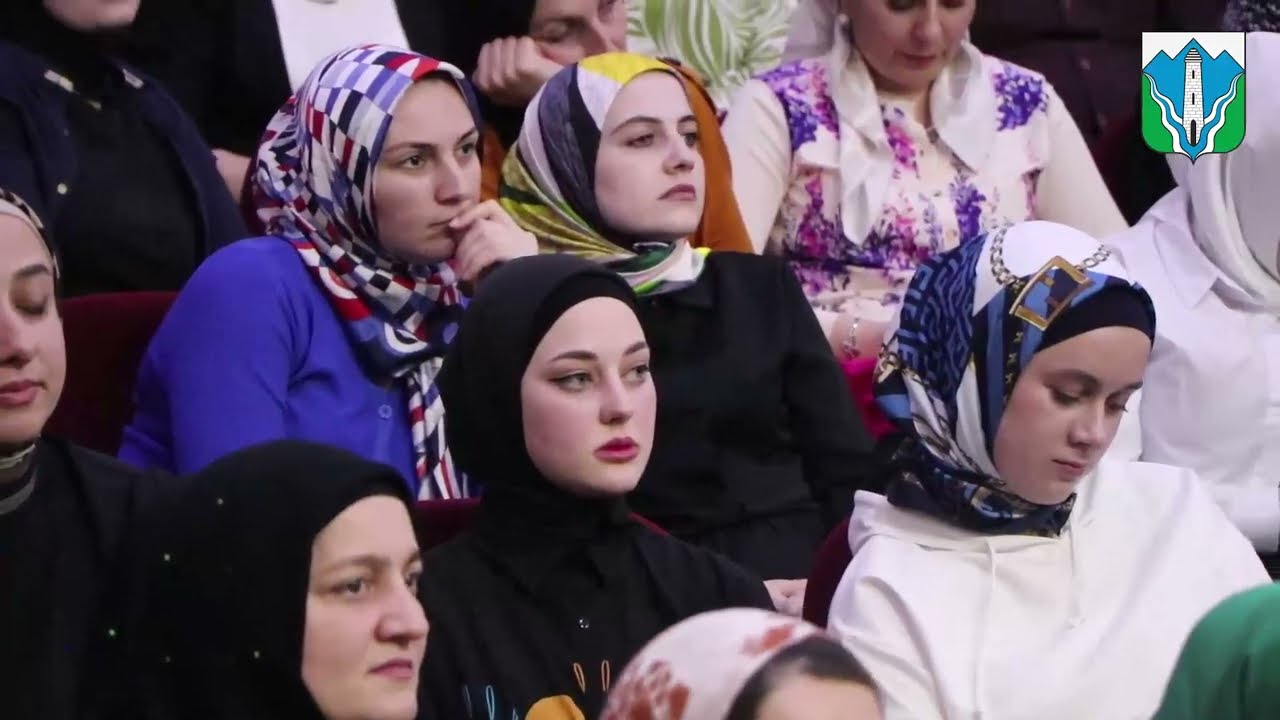The photograph captures a diverse group of women, all wearing Muslim-style headscarves, seated in several columns. Each woman's headscarf is distinct in color and pattern. In the bottom left, a Caucasian woman with a black headscarf and a touch of gray in her hair gazes forward. On the bottom right, a woman with a multi-colored headscarf in black, blue, and white is looking down towards her lap. Central to the image are two women sitting side by side; one covers her mouth with her hand, dressed in a blue shirt and a checkered-pattern headscarf, while the other wears a black shirt and a headscarf with yellow, white, and black hues, looking slightly upwards. To the right, a woman in a long-sleeve white shirt adorned with purple and pink flowers looks downward, her head not fully visible. Behind her is another person resting their head on a closed-hand. The women seem focused on an event occurring out of the frame. In the upper right corner, a brand symbol depicts a tall light yellow building, flanked by blue, squiggly lines representing rivers diverging and a blue mountain range in the backdrop. This image combines cultural elements and branding in a single frame.